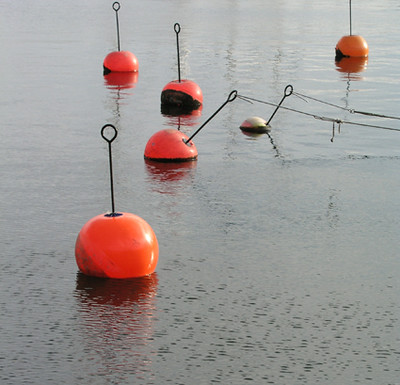The image depicts a serene, dark-colored body of water, likely a lake, characterized by its calm surface and subtle ripples. Central to the composition are several bright orange spherical buoys, analogous to upside-down lollipops, with their bottom quarters submerged and the rest floating. Each buoy is equipped with a long pole topped with a metal hoop for hooking or tying. The photograph, presented in a square format and in color, captures a tranquil scene devoid of bright reflections, suggesting an overcast day. In the midground, two buoys are tethered with ropes angled to the right, hinting at an unseen attachment, possibly a boat just outside the frame. The arrangement of buoys spans from the foreground to the background, creating a sense of depth in the otherwise still and placid setting.